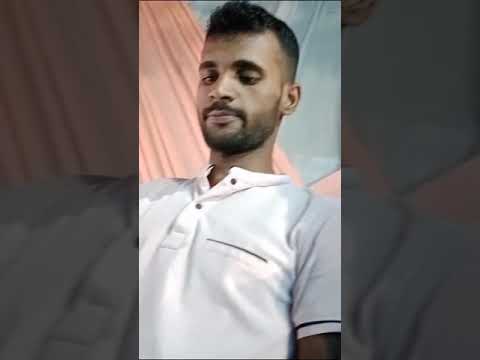The image features a three-panel composition, with the left and right panels darkened and containing zoomed-in portions of the central image. The central image is brighter and shows a close-up of a man from a slightly low angle, suggesting a selfie-like perspective with the phone positioned below his face. The man, who appears to be Hispanic, has a short curly black haircut and sports a black goatee and mustache. He is wearing a white polo shirt with short sleeves, which have black bands around them, and his facial expression is neutral, possibly contemplative, as he gazes downward.

The background features two intersecting sheets - a pink one on the left and a white see-through drape on the right, which form a V-shape around his head. There is also a hint of a cloudy, blue background behind the drapes. The zoomed-in sections on either side match the original image, each focusing on one of his shoulders, creating a cohesive frame for the central picture. This image appears to be a still from a social media post, artfully encapsulating the man's thoughtful demeanor amid a softly colored backdrop.